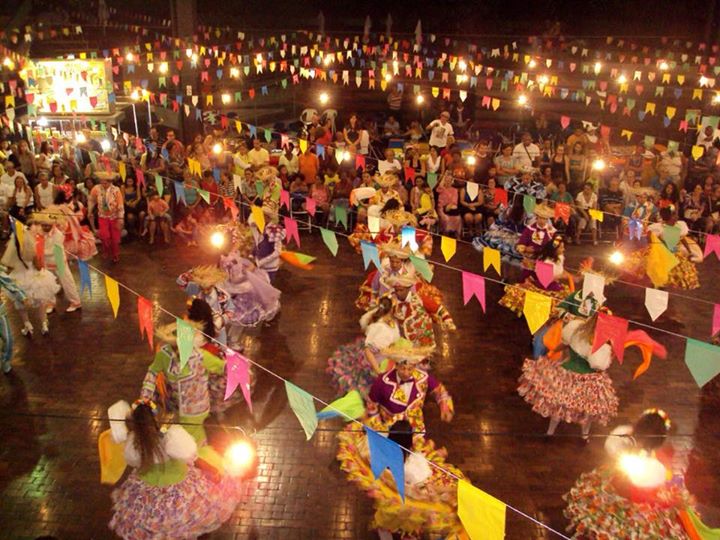Captured from a bird's-eye perspective, this vibrant image portrays a festive dance party, potentially of Mexican or Indian origin. Multicolored streamers adorned with small flags in hues of blue, green, and pink drape across the scene, creating a canopy of color against the night sky. Below, a brick dance floor serves as the lively stage where columns of people, predominantly women in voluminous, floral dresses, showcase their rhythmic movements. At the top of the picture, rows of seated spectators observe the celebration, their figures dimly lit against the darkness beyond the dance hall. String lights with glowing bulbs illuminate the dancers and enhance the festive atmosphere, capturing the essence of a culturally rich night of dance and merriment.